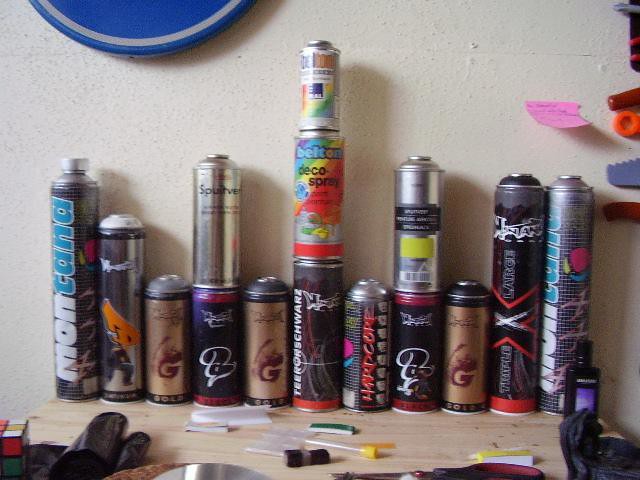This image captures a cluttered tabletop scene featuring several types of spray paint cans. The light wooden table, small in size, is cluttered with miscellaneous items including a roll of trash bags, a pair of scissors, and a Rubik's Cube in the bottom left corner. The spray paint cans are arranged closely together against a white, textured wall, some even stacked in multiple layers. Among the cans, one prominent tall purple can features the word "Montana" in white and blue font, and it still retains its cap. There are also three brown cans with gold labels and red 'G' logos at the bottom, identified as Gold, and a distinctive gray can. A silver can is positioned centrally, and another can marked with "Belton Deco Spray" flaunts a colorful rainbow design. Above, part of a blue circular wall hanging peeks into the frame, and a pink post-it note sticks to the right side of the wall. This assortment of vibrant cans, set against an ivory backdrop, creates a visually intriguing yet chaotic scene.